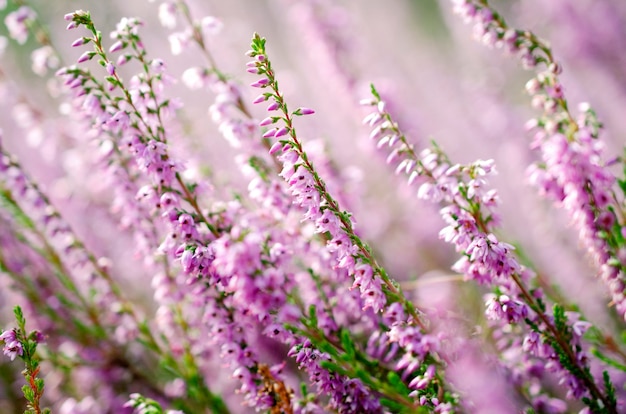This horizontally aligned rectangular close-up image showcases a collection of tall stems with light purple flowers accented by dark purple centers. Emerging from the lower right and angling towards the upper left, the stems are brown with tiny green leaves and scattered small dots that resemble leaves. Some flowers at the bottom of the stems have fully bloomed, displaying their elegant light purple petals with distinct dark centers, while those at the top are still budding, appearing as pointed tips. The image's blurred background, created by a bokeh effect, features similar flowers, enhancing the focus on the clear and detailed flowers in the foreground. The delicate contrast of the light purple petals against the green and brown stems creates a visually enchanting nature scene.